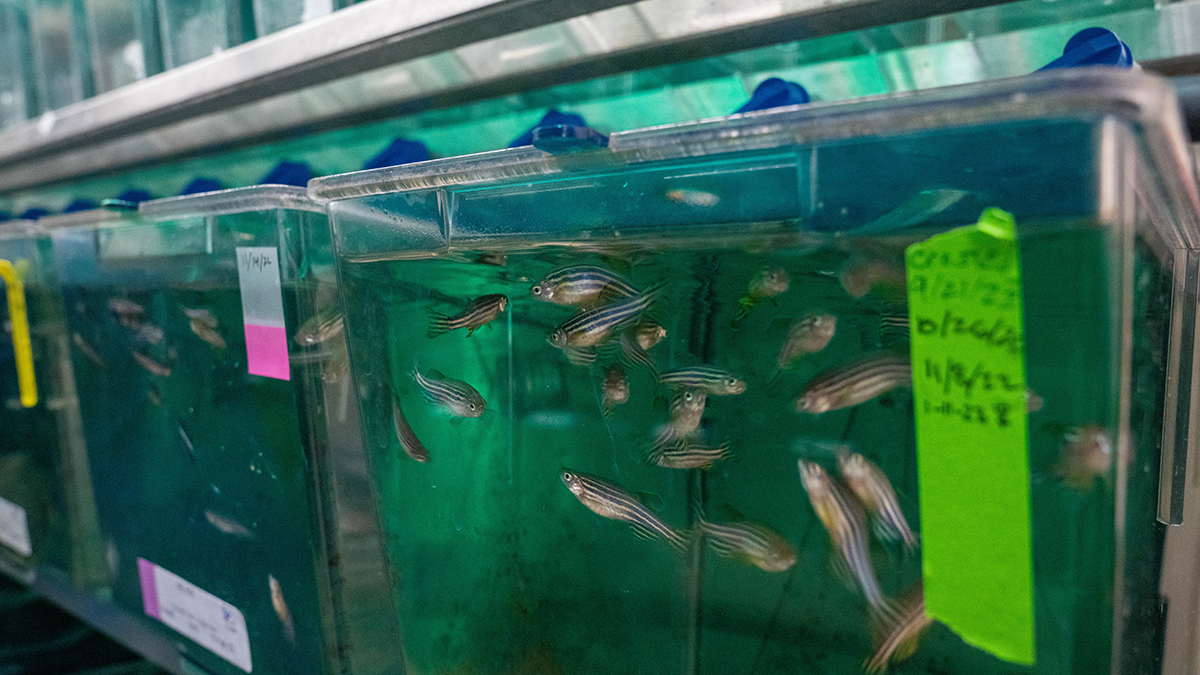This photograph, taken inside a commercial fish shop such as a Walmart or local pet store, showcases a fish tank filled with approximately 15 to 20 small, long, minnow-style fish with translucent gray bodies and distinctive black and white stripes. The fish appear to be swimming in somewhat dirty, bluish water, highlighting the possibly inadequate tank maintenance. The plastic tank is front and center in the image, featuring a lime green piece of tape with dates written on it that are hard to read due to the overall out-of-focus quality of the image. In the background, towards the left, two other tanks are partially visible, marked with pink and yellow labels, respectively, although they are also out of focus. Above these tanks, there are additional shelved containers and some kind of metal ledge. The image heavily suggests a commercial setting where these small fish are likely for sale.